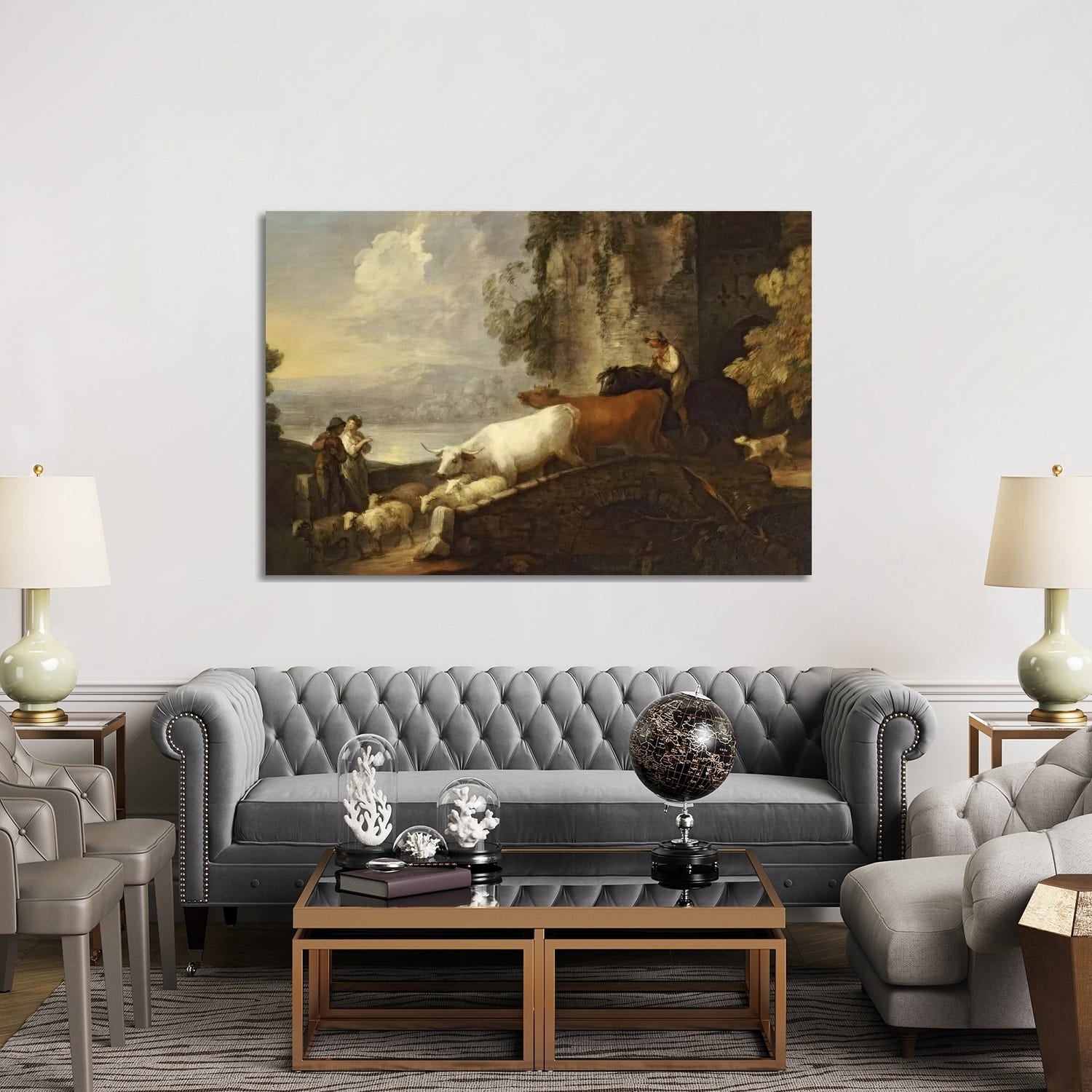This photograph captures a meticulously arranged living room, showcasing both vintage charm and contemporary elegance. Central to the room is a large, velvet tufted gray sofa, flanked by two pewter-colored leather chairs on the left and a single, plush, gray armchair on the right, adjacent to a modern side table. The furniture is oriented around a prominent brown coffee table with a glass top, adorned with a few tasteful decorations: a globe, a book, and glass dome enclosures containing delicate white coral or flowers.

On either side of the sofa stand two chrome and glass end tables, each topped with a white lamp featuring a white shade. The room's focal point, however, is the grand canvas mounted above the sofa on the expansive white wall. This screen print of a classical painting portrays a pastoral scene: two women conversing in a field, accompanied by cows crossing a bridge, sheep nearby, a dog in the background, and possibly a horse and rider herding the animals. The scene is set against a muted sky with a hint of an Italian town or building in the distance, surrounded by trees. This elegant and thoughtfully designed space harmonizes both modern and traditional elements, creating a warm and inviting atmosphere.